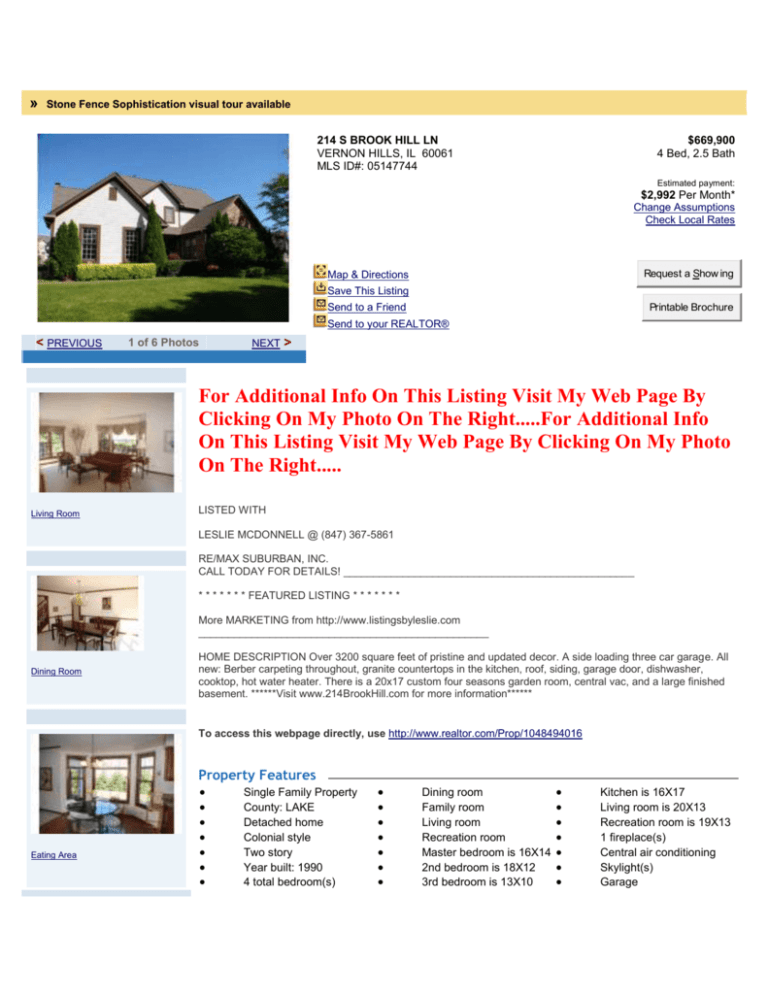A beautifully designed promotional image for a property listing. The image features a white background with a striking yellow header. At the forefront is a captivating photograph of an elegant house painted in white and brown. Prominently showcased is the address "214 S Brookhill Lane" and key details highlighting the home’s appeal: 4 beds, 2 baths. The image also includes navigational cues, offering a visual tour with an option to view “previous” or “next” photos (one of six total). For more information, the image directs viewers to visit the agent's webpage by clicking on their photo to the right. The property is listed with Leslie McDonald, whose contact number is clearly displayed as (847) 367-5661.